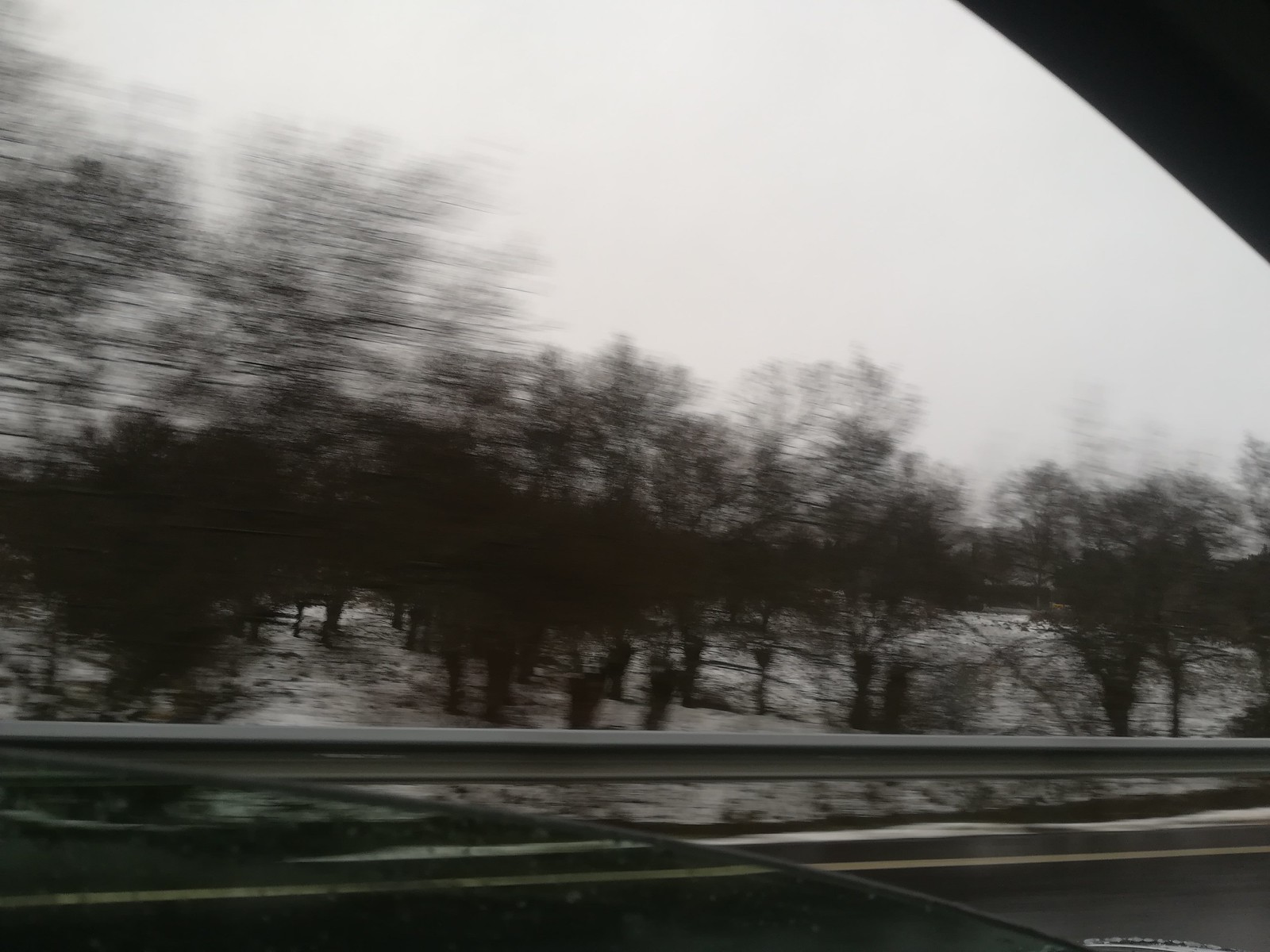In this hauntingly monochrome photograph, likely an old black and white image with a greenish tint, we peer through a car window revealing a dreary highway scene. The lower left corner of the frame captures the edge of the window, hinting at the viewer's perspective from inside a vehicle. Just beyond the window's edge, the pavement is visible along with a yellow street line marking the divide of the road. Dominating the midsection of the photograph is a large, gray metal guardrail that stretches horizontally across the frame, a steadfast barrier separating the highway from the surroundings.

Beyond the guardrail, the terrain slopes upward in a small snow-covered embankment dotted with trees, their forms blurred and indistinct, contributing to the image's moody atmosphere. The backdrop of the scene reveals more trees standing in solemn alignment, their presence softened by a blanket of snow. Overhead, the sky is overcast, the dense gray clouds adding to the somber ambiance, suggesting the scene is either amidst a snowfall or simply during a very overcast, gloomy day. The top right corner of the picture includes the metallic chassis of the car door, emphasizing that this entire glimpse into a wintry roadside landscape is framed from within the vehicle.